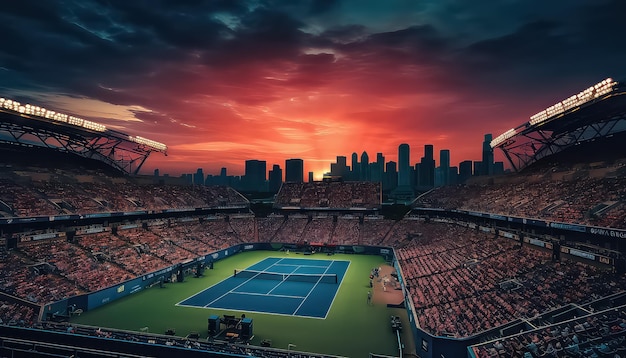The photograph depicts a surreal, heavily-edited scene of an outdoor tennis stadium. The rectangular tennis court itself is primarily green with distinct white lines segmenting various areas of play. Central to the court are two black posts holding a black and white net. Surrounding the court is a white and green border, beyond which lies a low blue wall separating the spectator seating areas from the court. The stadium seating is multilevel, filled with red chairs, and occupied by multiple spectators, some of whom are also standing on the green section of the court, suggesting an impending tennis match.

The background features a cityscape with looming skyscrapers, giving a grandiose feel to the environment. The sky above is painted in dramatic hues, transitioning from an orange-reddish light near the setting sun to darker tones of gray and black further up, creating a stark contrast with the scene below. The lighting throughout the image gives an artificial, almost painting-like effect, with plenty of brightness and clarity, highlighting the unnatural ambiance of the entire setting.